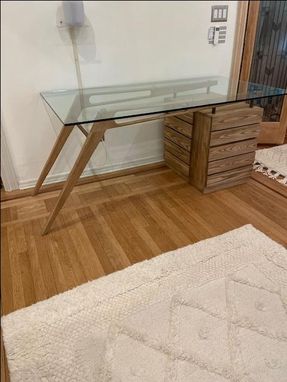The image depicts a room with caramel-colored wood floors and a modern, minimalist design. In the foreground, there is a white, fluffy area rug featuring a diamond pattern created by different tufting heights. The rug contrasts against the wood floor. Against the far wall, there's a glass-top desk with a mid-century modern aesthetic. Its design includes thin, angled wooden legs on the left and a sturdy wooden frame on the right, which is a block-like structure with drawers and is supported by four metal posts. Behind the desk on the beige wall, there's a gray cylindrical light fixture mounted above it. To the right of the desk, towards the upper right corner of the image, a door with a wooden frame and frosted, decorative glass is visible, along with a light switch. Near the door, a small segment of another rug can be seen on the floor. The room is accented with brown trim along the base of the walls, enhancing its classic-modern blend.